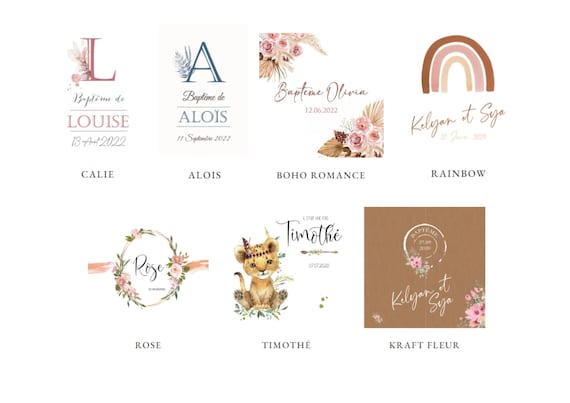The image showcases a series of seven greeting cards, displayed on a solid white background, arranged in two rows with four on the top and three on the bottom. Each card features a distinctive logo and design, primarily in cursive and serif fonts, with French text labels and floral motifs being prominent.

Starting from the top left, the first card displays a red capital "L" with floral patterns, titled "Baptism du Louis," dated 14th April 2022 in Calais. The next card features a blue "A" with leaf designs, labeled "Baptism Day Alois," dated 11th September 2022 in Alois. The third card is named "Baptiste Oliva," dated 12th June 2022, with bouquet designs on the corners, identified as "Boho Romance." The fourth card in the top row showcases a muted rainbow pattern in brown, pink, and orange hues, titled simply "Rainbow."

On the bottom row, the first card displays a flower wreath design and is named "Rose." The second card features a golden-yellow baby lion wearing a birthday cap, surrounded by green plants, and is labeled "Timothy." The last card on the bottom right depicts a brown background with floral patterns and text that reads "Craft Flutter." 

These cards blend intricate designs with personal touches, creating a visually appealing collection suitable for various celebratory occasions.